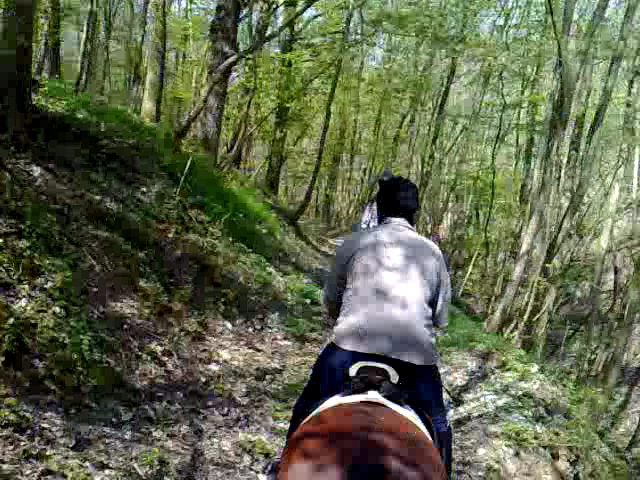The photograph is taken from the perspective of someone on horseback, capturing the view from behind of another rider ahead. The rider in front is sitting on a brown horse, wearing blue jeans and a gray long-sleeved shirt, appearing slightly uncomfortable. Only the horse's back and saddle are visible, with the rider's head tilted slightly to the left, suggesting a jostling motion as the trail winds through a lush, green forest. The trail itself is wooded and covered in leaves and wood chips, and the surrounding dense trees create a shady canopy. To the left of the trail, there's a rocky hill covered in moss and green vegetation. The scene also hints at another person in front of the visible rider, though they are not clearly seen. The horse's saddle features silver and black accents, adding to the detailed imagery of a serene forest trail ride.